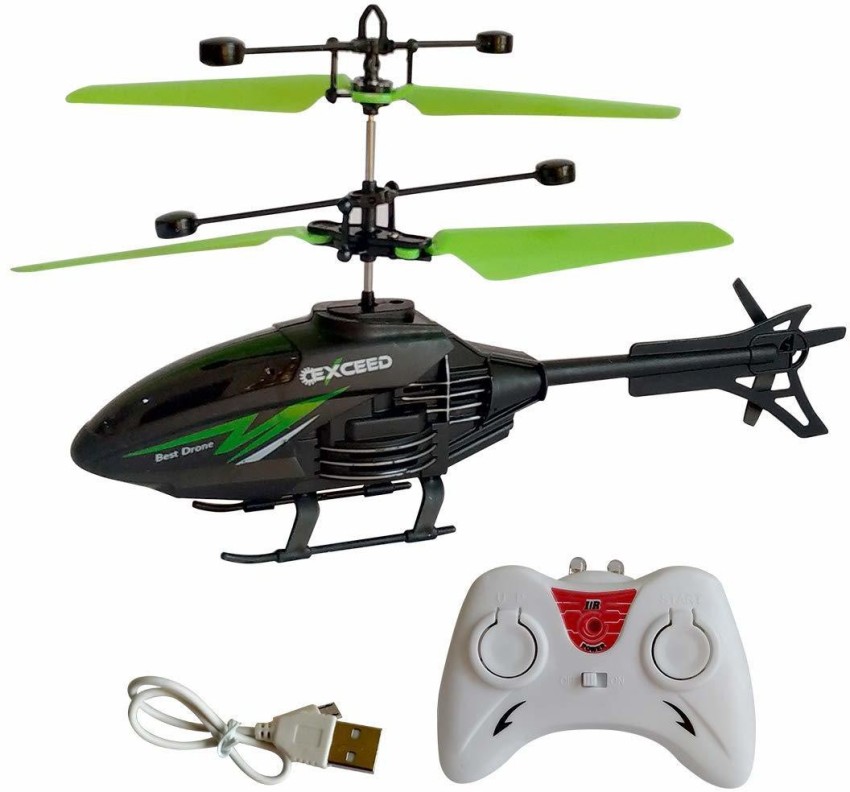The image showcases a remote control helicopter set against a stark white background. The helicopter, situated at the top, features a sleek black body accented with green propellers arranged in two layers. Prominently displayed on its side are the words "Best Drone Exceed." Below the helicopter, in the bottom left corner, lies a white USB charging cable. Adjacent to the cable, in the bottom right corner, sits a white controller adorned with a distinctive red sticker in its top middle section. The controller includes various buttons, with "on/off" at the bottom and "start" at the top right, suggesting intuitive operation. The detailed arrangement and clean background emphasize the product's sleek design and functional components, hinting at its retail readiness.